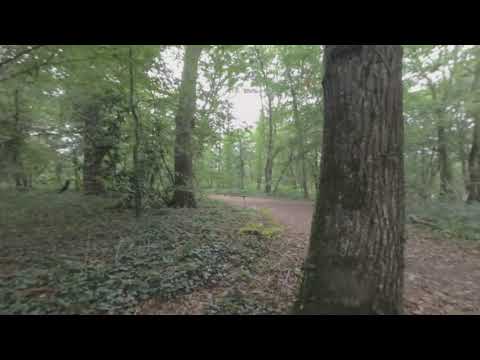This image depicts a serene woodland scene featuring a red soil path that meanders through a dense array of trees. The path bisects the scene, extending from the bottom right corner and leading into the lush greenery, with trees flanking either side. The soil appears distinctive in its reddish hue. Overhead, the sky is visible through the canopy, presenting a hazy gray or white appearance. The trees vary in their attributes; towering ones dominate the scene, accompanied by skinnier trunks reaching skywards. Surrounding the path are smaller plants, leaves, and occasional patches of greenery, but not in abundance. Nestled at the base of a prominent oak tree in the foreground, the scene provides a view of its rough bark texture. In a slightly blurry detail to the left, there might be a black dog or another dark creature, adding a hint of mystery. The overall framing of the image resembles the aspect ratio of a high-definition television, slightly wider than it is tall, with dark black borders accentuating the upper and lower edges. The setting suggests a calm, autumnal atmosphere, although the foliage is sparse, contributing to the tranquil ambiance of the picture.